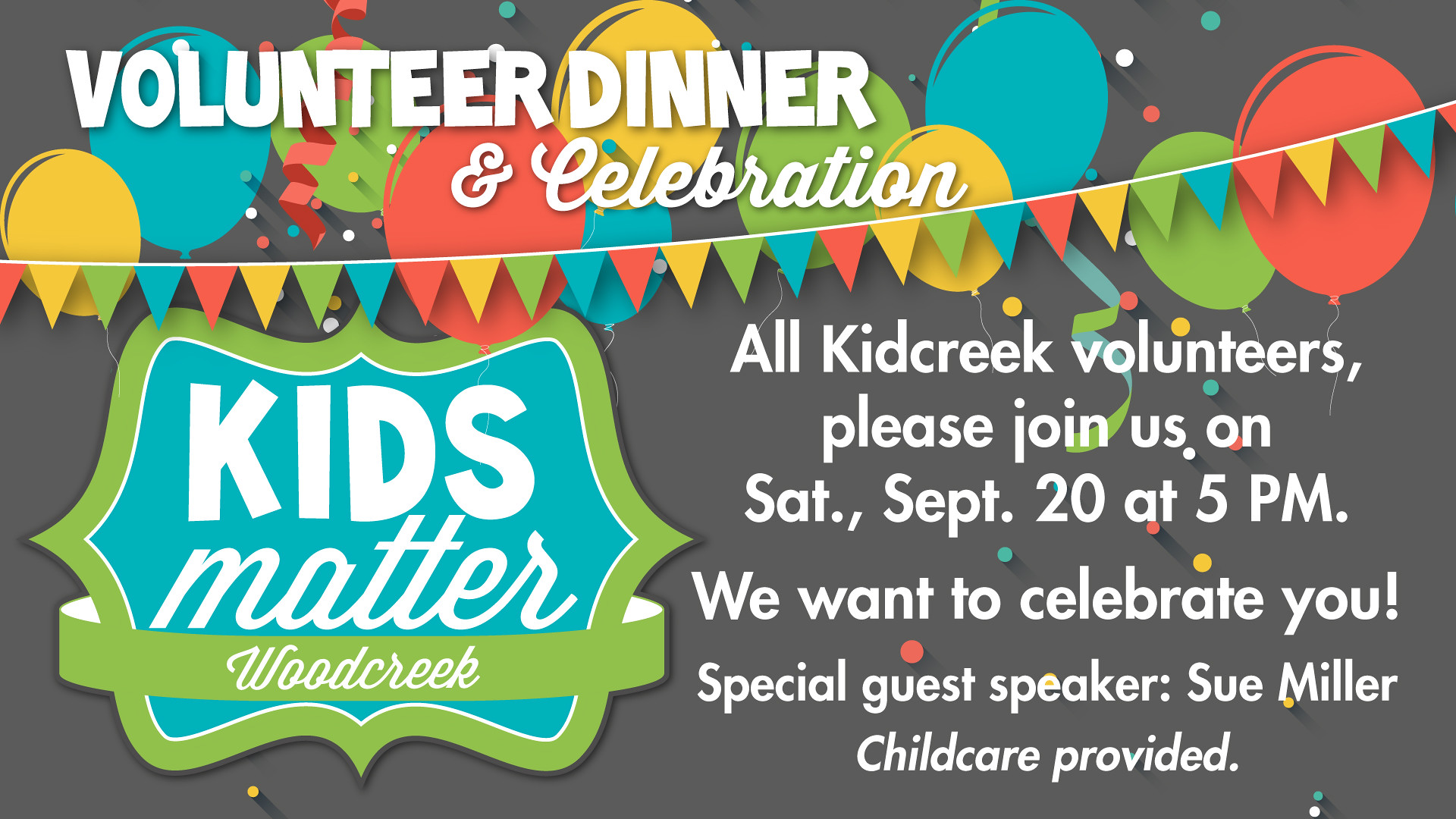This digital ad, displayed in landscape orientation, invites all Kid Creek volunteers to the Volunteer Dinner and Celebration hosted by Kids Matter Wood Creek. The event is scheduled for Saturday, September 20th, at 5 p.m., promising a festive evening complete with a special guest speaker, Sue Miller. Child care will be provided, making it convenient for families to join. The ad features a vibrant design with a black background and a decorative banner of pennants in blue, red, yellow, and green stretching across the top. These colors are echoed in the multicolored balloons and streamers scattered across the image, adding to the celebratory atmosphere. On the bottom left, a green and blue logo in a shield formation prominently displays "KIDS MATTER" in bold white letters and "WOOD CREEK" in white script on a green banner. Basic gray dots in the background add subtle texture, enhancing the overall design without overpowering the colorful elements. This cheerful and inviting ad effectively communicates the event details and the welcoming spirit of the celebration.